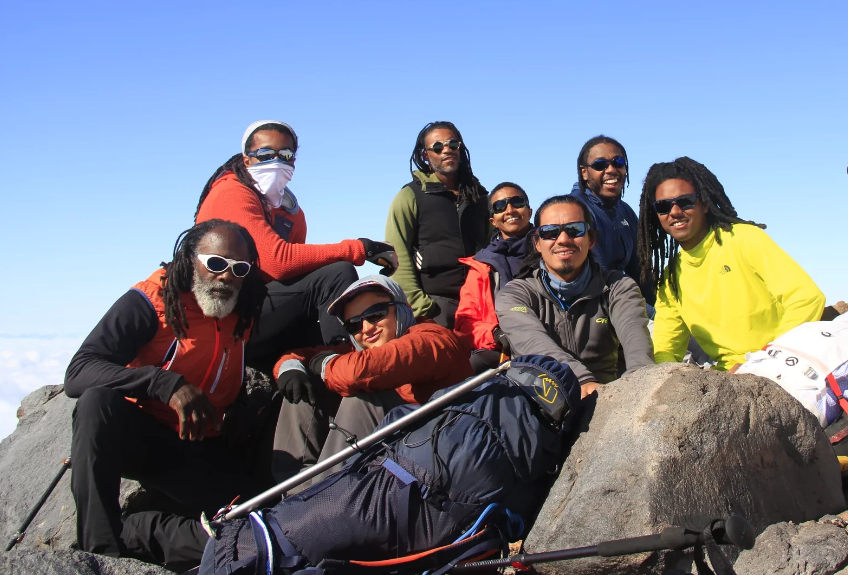In this captivating image, a diverse group of eight mountain climbers pose for a picture atop a rugged, large gray-brown rock formation. Against the vibrant backdrop of a clear blue sky with sparse clouds, these adventurers showcase a variety of colorful outdoor attire and gear, indicating a potentially chilly yet sunny environment. All clad in long sleeves, they are equipped with sunglasses to counter the bright sunlight. Notably, they display a mix of red, green, gray, black, and blue clothing, with some layered in vests and jackets, and one individual wearing a mask covering the lower part of their face—hinting at the cold or perhaps for dust protection.

On the left, one climber is crouched down, sporting a black jacket, red vest, black pants, and striking white sunglasses, his black hair braided and accompanied by a gray beard. Just above him stands a man in a red shirt, black pants, a white hat, and a white face scarf. To his right, another climber in a green shirt and black vest with golden-rimmed sunglasses and braids wears gray pants. Central to the photo, a person with a red baseball cap, a layered gray and red hoodie, and gray pants smiles warmly, standing in front of a blue holder containing a wrapped sleeping bag or tent.

To the right of this central figure is a man in a gray jacket over a blue shirt, donning black sunglasses and short black hair. Behind him and slightly leaning in between the man in green is another smiling climber, dressed in dark blue with short hair, sunglasses, and a red jacket. Lastly, two more individuals on the far right, both with braids and sunglasses, are visible; one wears a yellow-green jacket and the other a dark green jacket, the former standing next to a white bag.

Their expressions vary, with most smiling, showcasing the joy and camaraderie of their adventure stop, as they rest and possibly refuel before continuing their climb. The scene vividly captures the essence of their spirited outdoor journey.